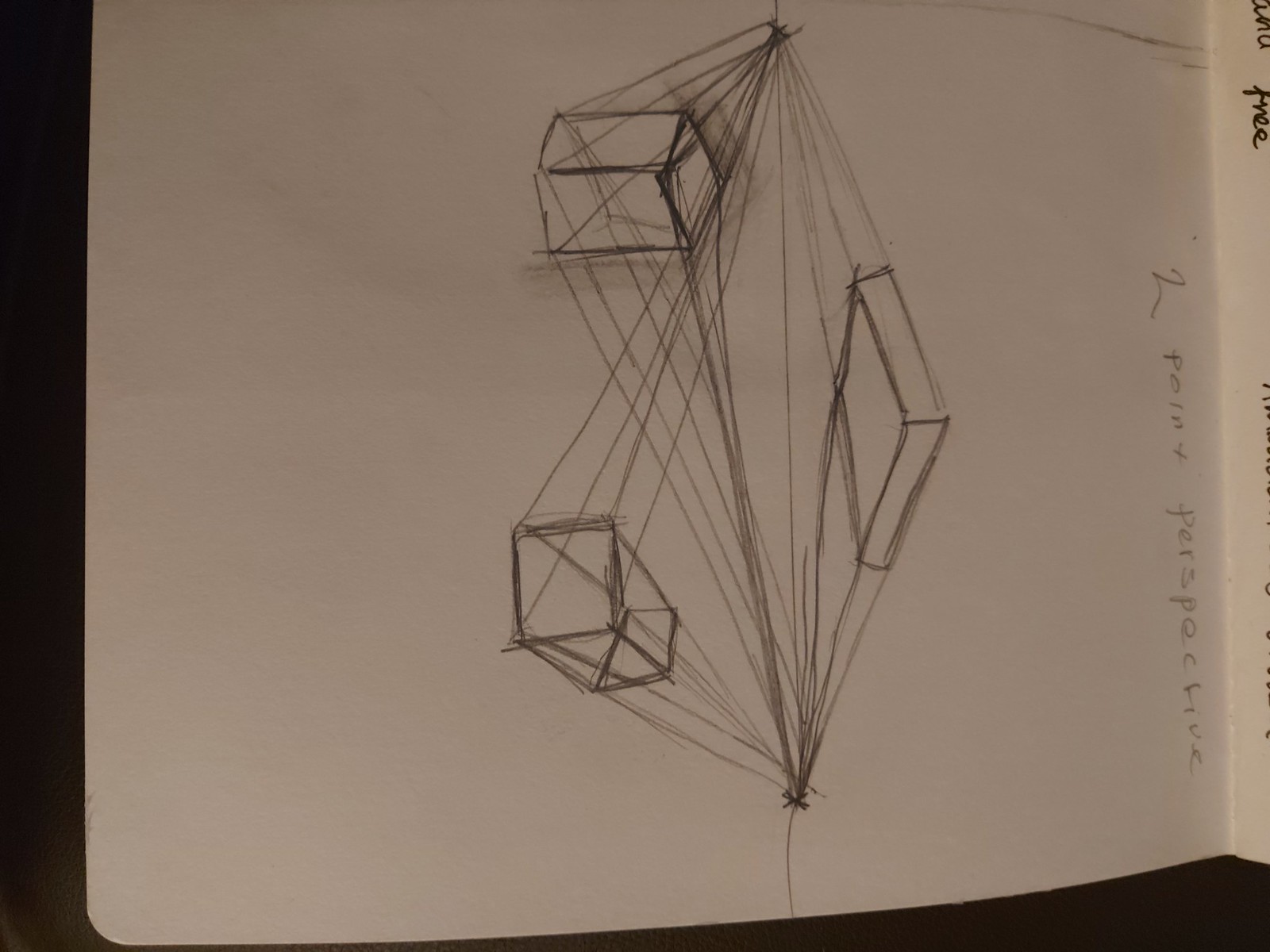An indoor color photograph showcases a minimalist pencil sketch on a white sketchpad. The central focus is a diamond shape, with its left point slightly notched and the words "Two-Point Perspective" vertically printed to its immediate right. The drawing features lines originating from the top and bottom center of the diamond, fanning out diagonally to both the left and right sides. Notably, to the right of the center, a small diamond shape can be seen, contributing to the overall geometric composition. On the left side of the sketch, two three-dimensional rectangular objects are depicted—one positioned in the lower part of the sketch and the other in the upper part, with a triangular wedge notched between them. Lines extend from these triangular points towards the central bottom point of the diamond, converging where all the radiating lines meet. Similarly, a few lines extend towards the top. The sketch, rendered solely in pencil, is rudimentary and consists of approximately 50 to 60 lines. The background around the sketchpad's edges is black, particularly evident at the far left and lower right corners of the image.